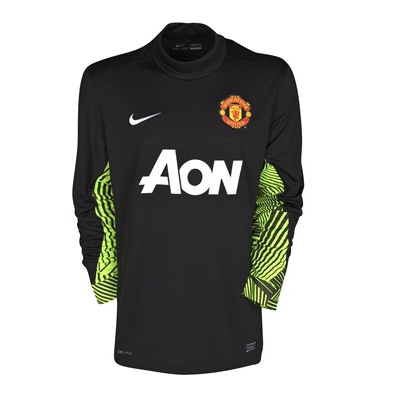The image features a black, long-sleeve jersey with green stripes near the ends of the sleeves, displayed against a white background. The shirt has a high, circular collar and a sleek athletic design. The right chest area displays the iconic white Nike swoosh symbol. Across the chest, the letters "A-O-N" are prominently printed in white. On the left chest area, there is a circular emblem featuring a shield with red and yellow detailing. The overall presentation of the shirt is as if it's on an invisible model.